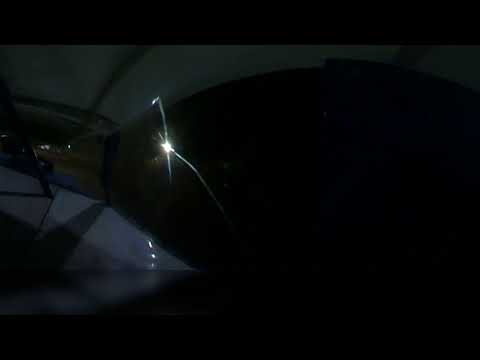In this dimly-lit, animated scene, the focus is on an outdoor setting shrouded in darkness, with a strong sense of mystery and obscurity. The image is predominantly black, making it challenging to distinguish specific objects. However, on the left side, a faint outline of a gray structure, possibly a metal frame or a tarp, is visible. This structure seems to support a very bright yellow light, which is likely emanating from an overhead light pole, casting rays that illuminates part of the scene. The light is positioned slightly to the left of center, creating a stark contrast against the dark surroundings and reflecting off an unspecified object below. The overall composition suggests the setting is possibly inside a covered boat or a similarly enclosed outdoor area. The scene is animated, with a cartoonish style, which enhances its ethereal and ambiguous quality.